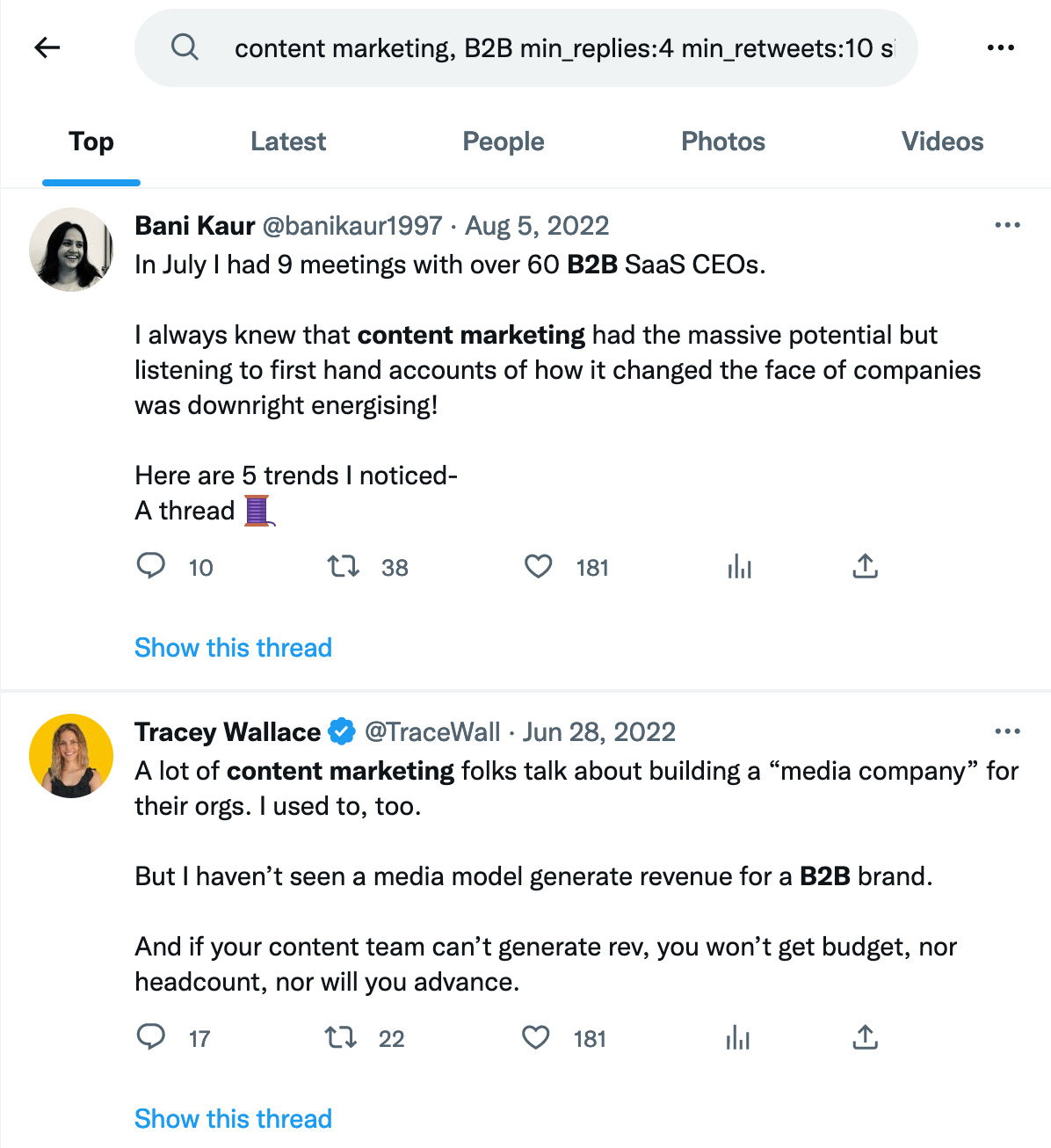A screenshot appears to be from Twitter, showcasing a search session with specific criteria in the search bar: "content marketing, B2B, min replies: 4, min_retweets: 10". The screen is partially cut off, ending at what may be the start of another word beginning with "S". At the top left are the back button and the 'more options' button, represented by three vertical dots. The top menu provides filtering options, including "Top," "Latest," "People," "Photos," and "Reviews."

The first tweet featured is from Banny Carr (@BannyCarr1997), posted on August 5, 2022. The tweet describes Banny's experience in July 2022, where she held nine meetings with over 60 CEOs from B2B SaaS companies. Banny expresses how witnessing the transformative impact of content marketing firsthand was invigorating and shares five observed trends in a threaded tweet, accompanied by a spindle emoji. This tweet has garnered 10 replies, 38 retweets, and 181 likes. Additional icons for analytics and sharing are visible.

The second tweet is from Tracy Wallace (@TraceWall) dated June 28, 2022. Tracy discusses the prevalent talk among marketing professionals about creating a "media company" for their organizations. However, Tracy posits that such a model hasn't been successful in generating revenue for B2B brands. She argues that if content does not produce revenue, it will not attract budget or headcount, nor will it foster professional advancement. This tweet has 17 replies, 28 retweets, and also 181 likes, along with icons for sharing and viewing analytics. Both tweets include a link to show threads at the bottom.